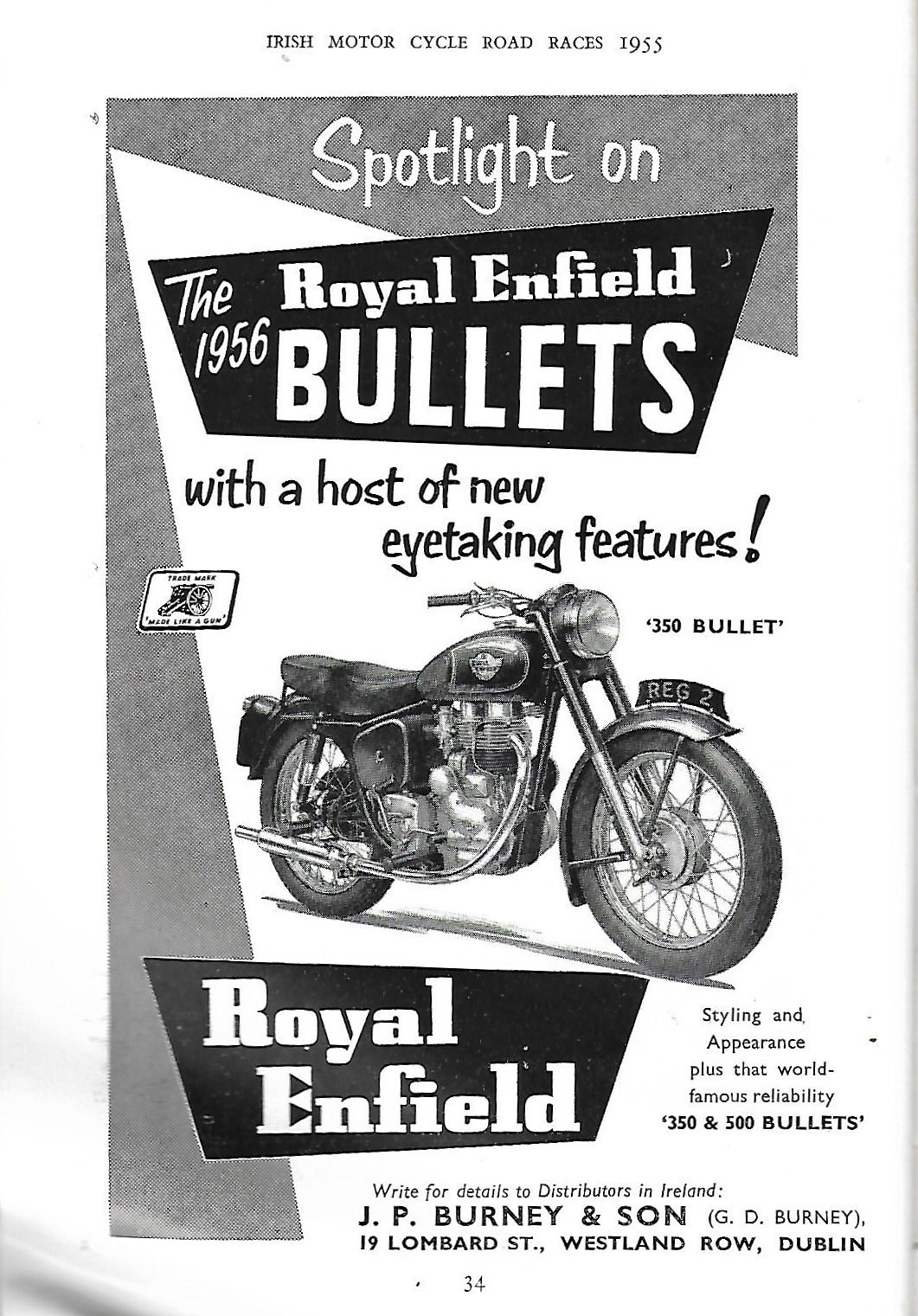The image is a black and white scan, possibly from a magazine or an advertisement flyer. The top of the page prominently reads "Irish Motor Cycle Road Races 1955," and it is noted as being page 34 of the publication. Below this heading, a large section highlights the "1956 Royal Enfield Bullets" with a description stating "a host of new eye-taking features." Dominating the central area is an illustration of a motorcycle labeled "350 Bullet," with the brand name "Royal Enfield" clearly indicated. Additional text emphasizes the bike's "styling and appearance plus that world-famous reliability," mentioning the availability of both "350 and 500 Bullets." The bottom of the page directs readers to "write for details to distributors in Ireland," providing the contact information for "J.P. Bernie and Son, 19 Lombard Street, Westland Road, Dublin."